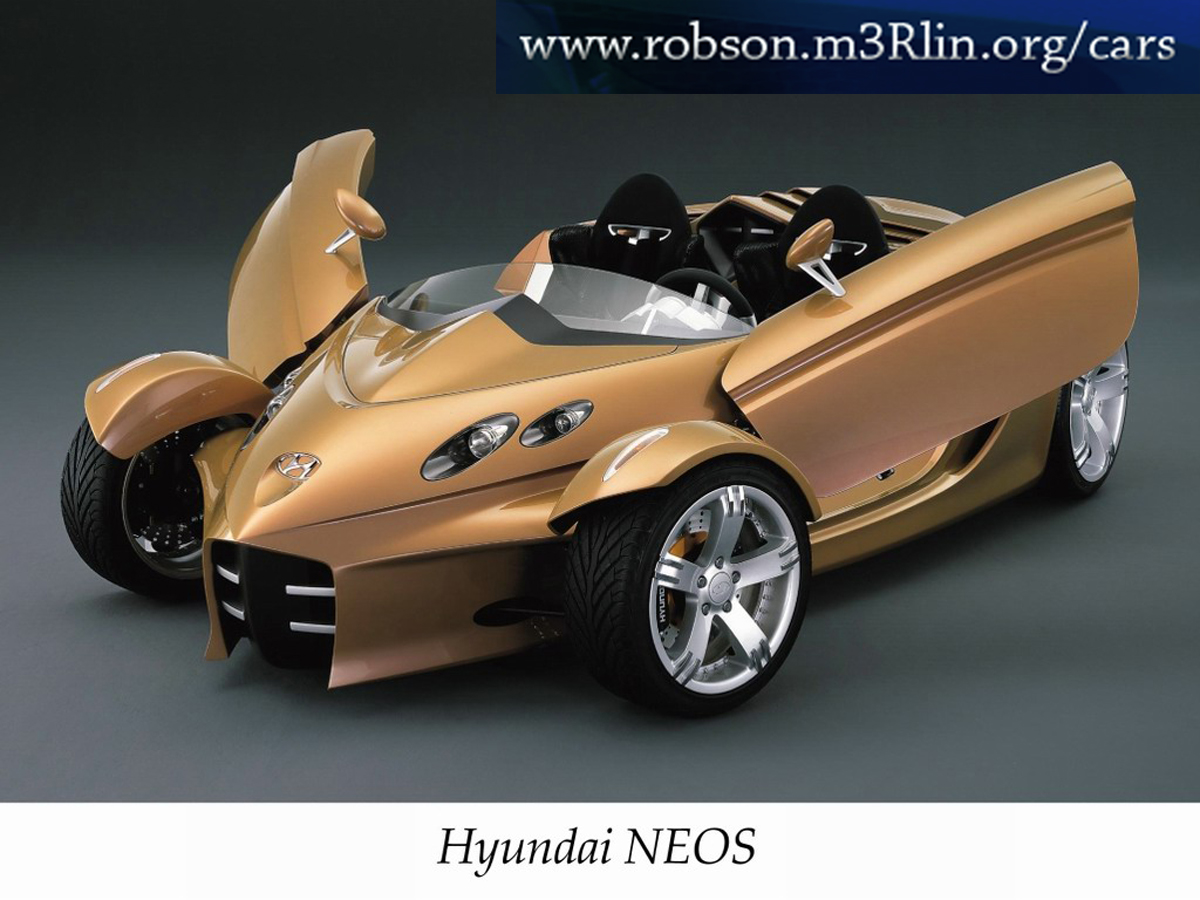The image portrays a detailed color illustration of a prototype Hyundai NEOS vehicle, prominently centered in a landscape orientation. The vehicle features a sleek, sporty design with vertically opening doors reminiscent of seagull wings. It sports a pointed front hood with a small black grille at the center, accentuated by two silver horizontal bars and the Hyundai emblem at the front. The car boasts large, jet black tires with chrome wheel rims. 

The image shows the car in a side profile with the vehicle angled toward the bottom left corner while its back faces the top right. The design includes black leather seats with a two-seater capacity, enhancing its futuristic, sporty appeal. The vehicle displays a palette of black, gray, white, peach, silver, and blue colors. At the top right corner of the image, there is a black horizontal band with a white URL that reads "www.robson.m3rlin.org/cars," and "Hyundai N-E-O-S" is captioned at the bottom. The illustration appears to simulate a showroom floor environment, possibly intended for a car dealership's website.